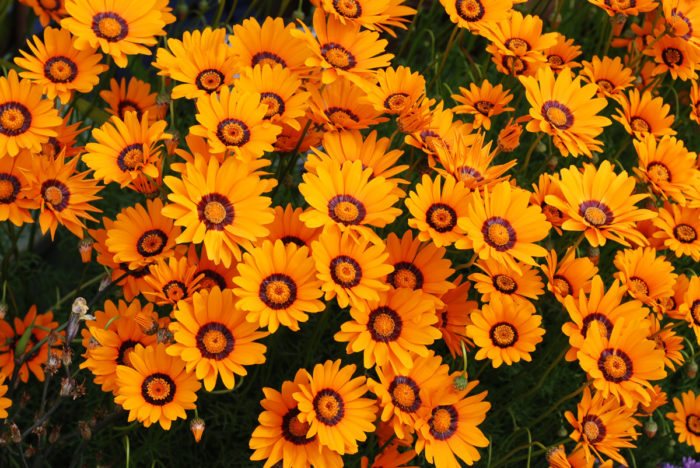This close-up photograph showcases a striking field of daisy-like flowers set against a very black background, emphasizing their vibrant colors. The flowers, viewed from above, manifest in a spectrum of yellow to orange petals. Their centers feature a captivating gradient, with a dark outer ring, a lighter yellow middle, and a red dot at the core. Among the fully bloomed flowers, a few buds are also visible, adding variety to the scene. The light green stems and subtle green foliage peek through, enhancing the floral composition. The darkness of the background amplifies the vivid colors, making this visually arresting photograph suitable for a nature site, floral showcase, or photo contest.